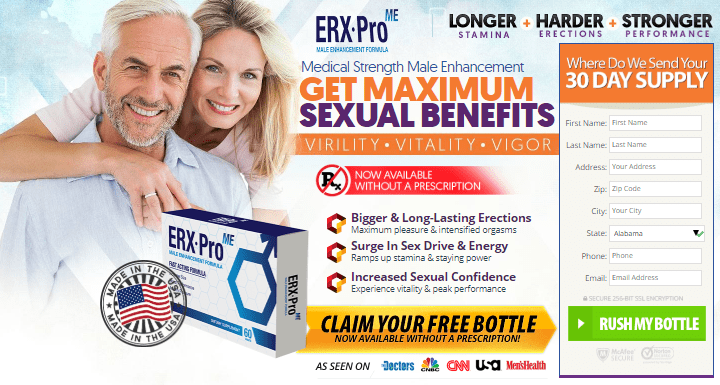In this advertisement for erectile dysfunction medication, we see an older Caucasian couple on the left side of the image. The man is wearing a light blue shirt and has predominantly gray hair, while the woman, who is dressed in a light pink shirt, has a hint of blonde and possibly some gray in her hair. Both have visibly white teeth and faces marked with wrinkles, showcasing their age.

In front of the couple, there is a box of ERX Pro-ME, characterized by its blue and white packaging. The box prominently features a circular "Made in the USA" logo, with a red, white, and blue American flag in the center. To the right of their heads, the product name "ERX Pro-ME Male Enhancement Formula" is displayed.

Adjacent to this, in bold black and purple text, the benefits of the medication are listed: "Longer stamina, harder erections, stronger performance." Below these claims, returning to the left-hand side next to the couple, there are additional assertions: "Medical strength male enhancement, get maximum sexual benefits—virility, vitality, and vigor."

Further down, a red banner announces that the medication is now available without a prescription, marked by a crossed-out RX symbol. Accompanying this are three red and orange octagon logos with thumb tabs emphasizing the product’s promises: "Bigger and longer-lasting erection, maximum pleasure and intensified orgasms, surge in sex drive and energy, ramps up stamina and staying power, increased sexual confidence, experience vitality and peak performance."

A yellow banner below invites viewers to claim a free bottle, reiterating its availability without a prescription, and mentions its feature on television with references to "The Doctors," CNBC, CNN, USA, and Men's Health. 

On the right-hand side, there’s a box with a purple banner asking, "Where do we send your 30-day supply?" There are fill-in boxes for personal information, including first name, last name, address, zip code, city, state, phone number, and email. At the bottom, a green bar labeled "Rush My Bottle" is visible.